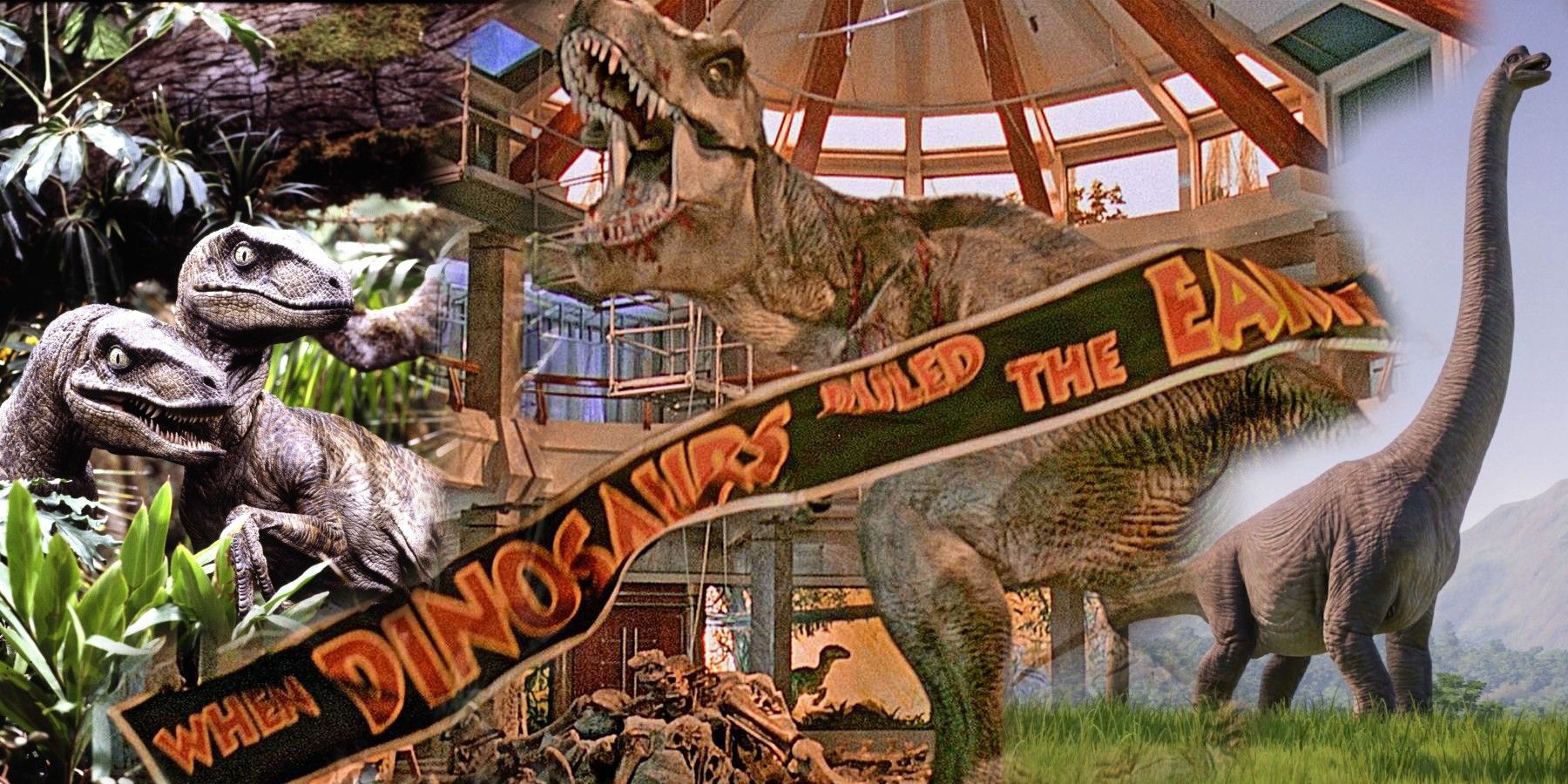The image is a detailed dinosaur poster set in what appears to be a museum-like domed enclosure. Dominating the scene, a gigantic, tan-colored T-Rex with its mouth wide open in a menacing roar stands centrally, with all its teeth visible, against a backdrop of foliage and plants. A black banner with red type outlined in dark orange runs diagonally from the left-hand to the right-hand corner, reading "When Dinosaurs Ruled the Earth," though the word "Earth" is somewhat obscured by the banner's bend. In the background, several other dinosaurs are present: a towering brontosaurus with its long neck craning upwards, an imposing triceratops, and a couple of gray dinosaurs on the left, one with its mouth partially open and the other with its mouth closed. Another dinosaur is faintly visible in the far distance. The setting merges elements of natural scenery, such as tall grass and a distant mountain, with man-made structures, including wood beams, scaffolding, a balcony viewing area, and large windows in the dome, through which the mountains are visible. The overall visual effect is a blend of animatronics and illustration, evoking a scene reminiscent of "Jurassic Park."